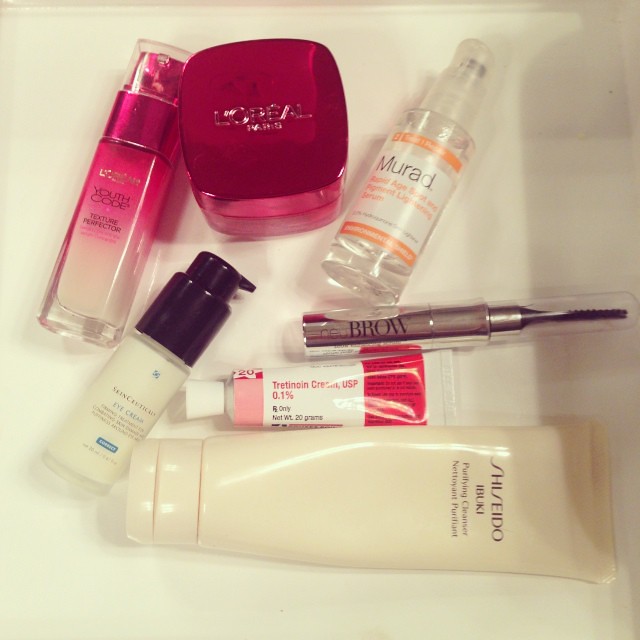This image features an array of diverse skincare products meticulously arranged against a pristine white background. 

In the upper left corner, a rectangular bottle with a clear body and a pink nozzle, capped by a transparent lid, stands out. The product, which hints at being some sort of foundation, bears the label "Youth Code."

To its right, a square-shaped box in a pink hue with a striking red lid prominently displays the brand name "L'Oreal." 

Adjacent to this, a clear spray bottle is slightly tilted to the right, featuring a white label accented with an orange band and the name "Murad."

Below this spray bottle, a brown, pencil-like object marked "brow" lies vertically. It is a brow shaping tool, equipped with a brush tip positioned to the right.

Returning to the left side of the image, there is a bottle oriented to the right, showcasing a black pump dispenser atop a clear container filled with a white substance.

Next to it, a tube of ointment with a white lid features a gradient design of pink, white, and red.

Just below this, a container lies horizontally with its lid to the left. It is an off-white tone and branded with "Shishito," indicating a premium skincare product.

This detailed arrangement showcases a variety of beauty and skincare essentials, perfectly displayed on a clean, white backdrop.